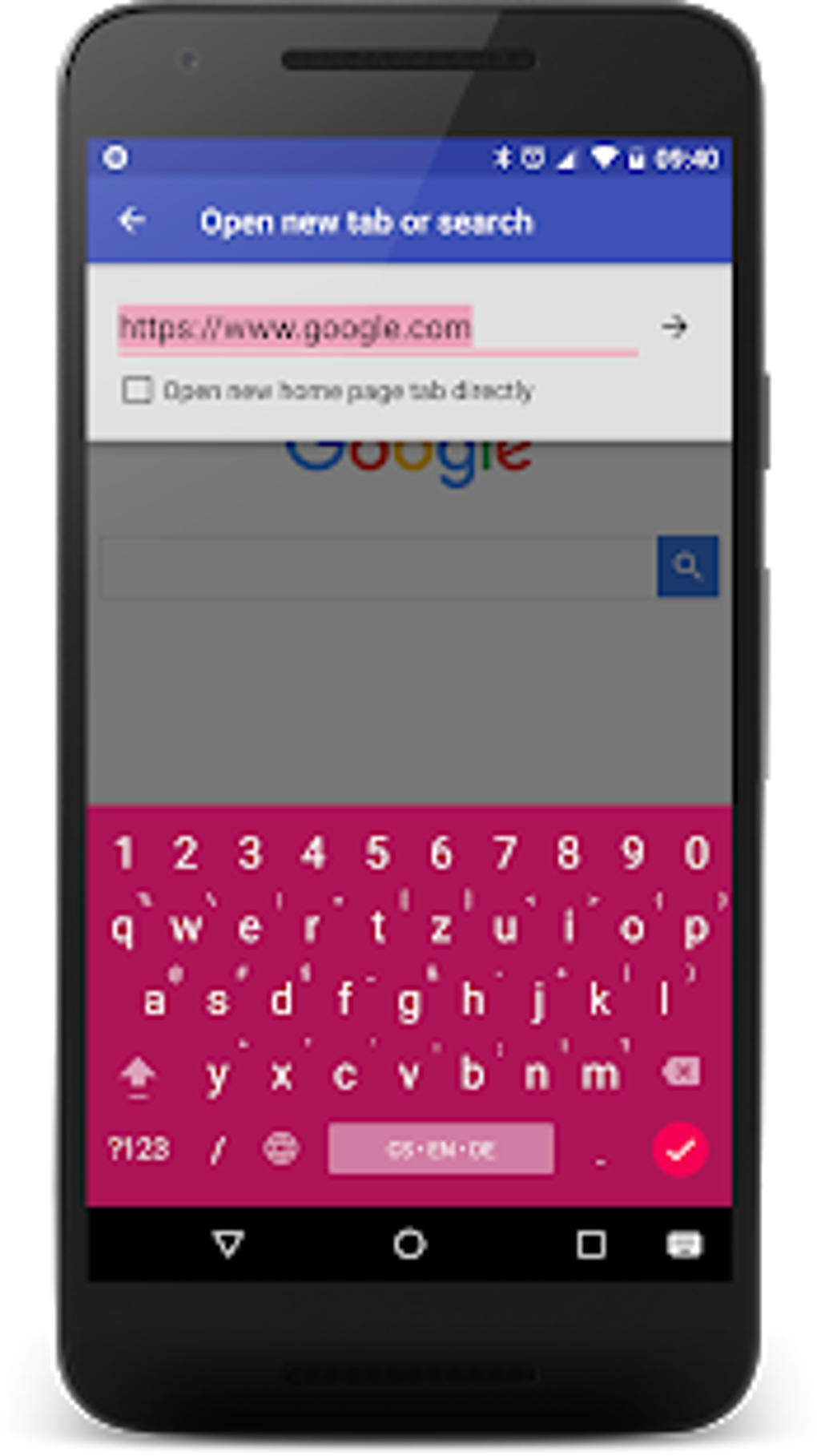The image displays a mock-up of an Android phone featuring a screenshot of an active web search within Google Chrome. The front of the phone showcases a typical Android smartphone bezel, but the screenshot displayed on the screen is noticeably blurrier, indicating it has been edited into place. The screenshot captures a moment where the user is interacting with the Google Chrome browser, evident from the inclusion of the browser’s address bar displaying "https://www.google.com" and an arrow pointing to a checkbox labeled "Open this homepage tab directly."

The keyboard is visible, demonstrating user input capabilities, and it is apparent that they have multiple global keyboards enabled, specifically labeled as EN (English) and DE (German). The keyboard itself is in a striking hot pink color. Below the keyboard are the standard Android navigation buttons: back, home, and recent apps (menu) buttons. The underlying screen shows the familiar Google search homepage, reinforcing the sense of an ongoing online activity within the browser.